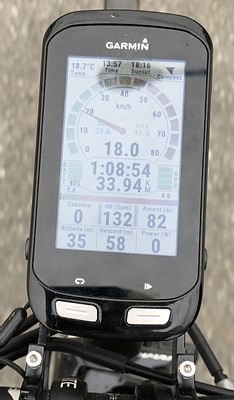This photograph features a sophisticated Garmin gauge, resembling a sleek, slim flip-phone, securely mounted on a bicycle. The device, encased in a black, rectangular frame, proudly displays the "Garmin" logo in small white text at the top. Its LED screen, although slightly obscured by outdoor reflections—including a noticeable reflection of a light pole—provides vital information to the rider. 

Centered prominently on the screen is a gauge, designed akin to a speedometer, with markings from 0 to 80 miles per hour. The needle and a digital display both indicate a current speed of 18 miles per hour. Directly below the speed readout, the display shows "108.54," likely representing the duration of the ride. Another figure, "33.94," is situated below the duration, possibly denoting distance traveled.

The background includes a partial view of the bike's front wheel, providing context and confirming that this gauge is used to monitor biking metrics accurately.